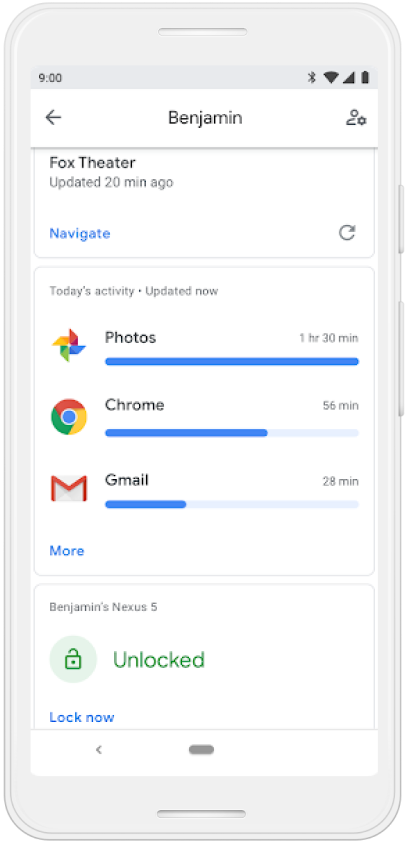The image depicts a white smartphone with various functional details visible on its screen. On the right side of the phone, hardware buttons for power and volume control are present. The phone also features a speaker at the top and a microphone at the bottom.

The screen displays multiple indicators at the top, showing the time (9:00), Bluetooth connectivity, Wi-Fi signal strength, and a full battery status. Below this status bar, the screen reads "Benjamin," with a dividing line underneath. To the left of "Benjamin" is a backward-facing arrow, and to the right is a profile icon depicted by a simple head and shoulders outline, accompanied by a settings symbol.

Further down, there's a section titled "Fox Theatre," which was updated 20 minutes ago. Within this section, the word "Navigate" is written in blue in the bottom left corner, and a refresh symbol (a circle with an arrow) is on the right.

Underneath, a separate box reads "Today's Activity," updated just now. This section includes the Google Photos icon (a pinwheel) labeled "Photos," with a completely full blue bar indicating "1 hour 30 minutes." Below that, the Chrome browser icon labeled "Chrome" shows a nearly three-quarters full blue bar, indicating "56 minutes" of use. Further down, the Gmail icon labeled "Gmail" displays a bar about one-third full, with "28 minutes" noted next to it. The word "more" is written in blue font below these entries.

At the bottom of the screen, another box is labeled "Benjamin's Nexus 5" with a slightly open lock icon next to it, signifying that the phone is unlocked, indicated by the text "unlocked" in green font. An additional instruction states, "you can lock now."